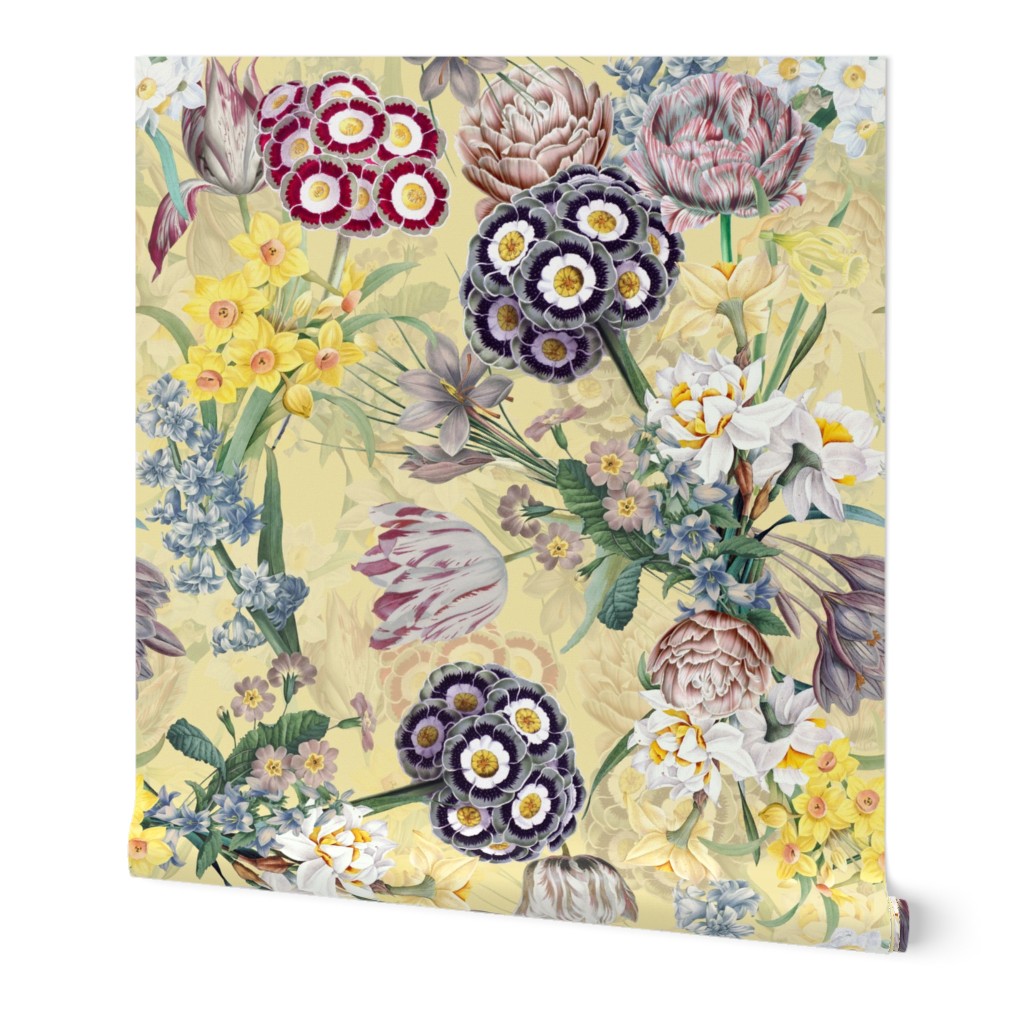Set against an entirely white background that eliminates any perception of edges, this image features a partially unrolled roll of wallpaper at its center. The wallpaper, which is depicted as if it were a digital product photo, showcases a vibrant floral pattern on a yellow backdrop. The design exudes a Victorian vibe and includes a variety of flowers: densely clustered green stems give rise to circular bunches in shades of purple, white, yellow, and red. Interspersed among these are singular, larger flowers in hues of pink and blue. Some flowers exhibit unique characteristics, such as black-ringed white petals, magenta replacements for the black, and six-petaled yellow blooms surrounding an orange center. Additionally, the pattern includes blue flower clusters and red and white wrinkly, striped flowers, all oriented in different directions. A subtle, staggered, lower-opacity repetition of the floral pattern fills out the background, enhancing the richness of the design.